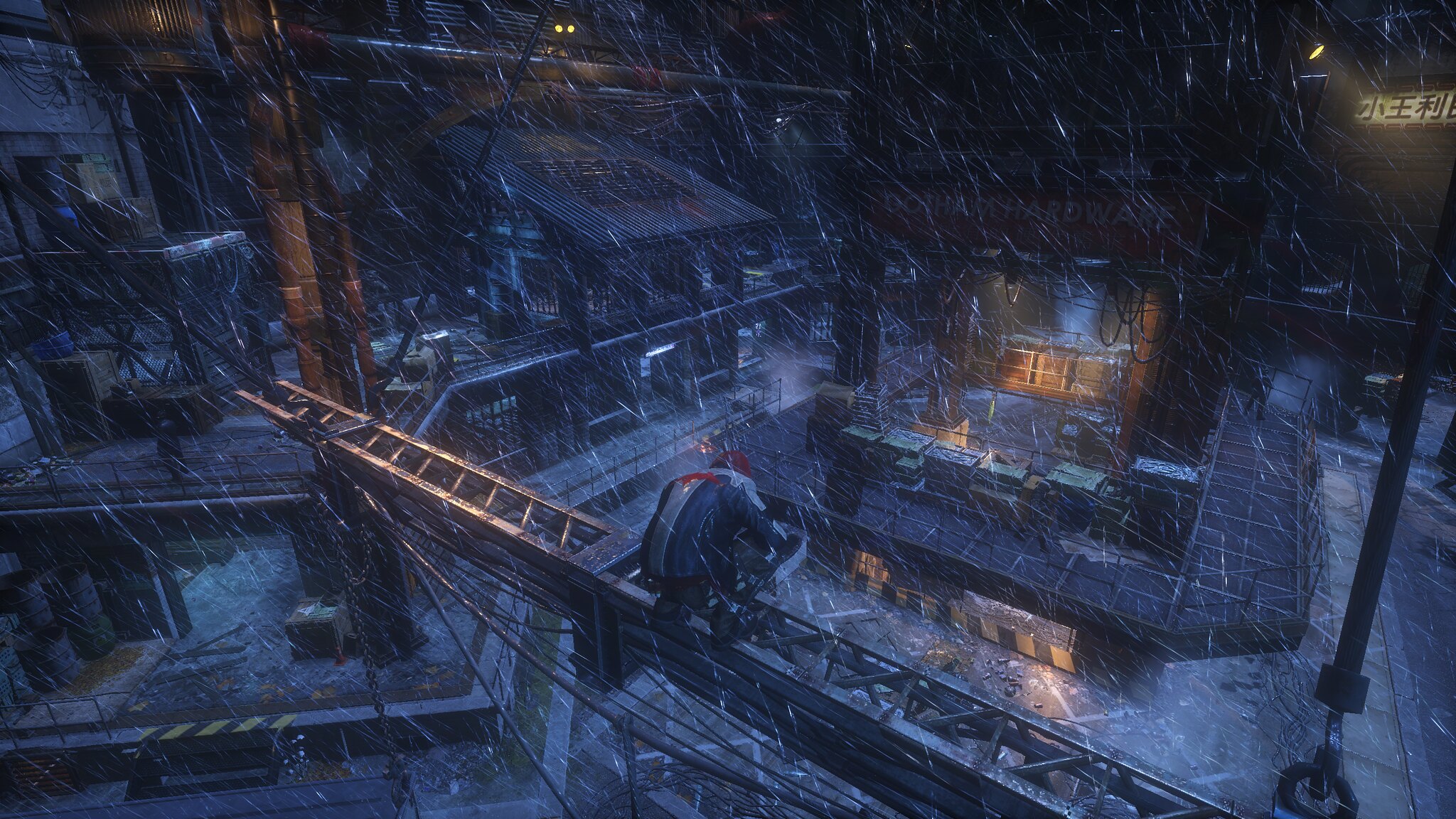In this highly atmospheric and sophisticated video game scene, a lone character crouches on a metal scaffolding, surrounded by the dark, rain-soaked ambiance of an industrial area. The scene appears to be taken at night, accentuated by the realism of the graphics, with thin lines of rain adding to the immersive experience. The protagonist, clad in a silver and blue long-sleeved jacket emblazoned with a logo, wears long pants, shoes, and a red cap. He is hunched over, carefully observing the area below from his precarious perch on the scaffolding, which extends from the lower right to the middle of the left side of the image. Through the crisscrossed metal grating, we glimpse various levels and platforms ahead, laden with stacked boxes and other indistinct objects. In the background, distant buildings with illuminated windows outline a sprawling, warehouse-like environment, suggesting an industrial park or similar setting. The meticulous detail and moody aesthetic suggest this is an intense moment in what might be an action RPG game, where the character navigates and oversees a complex, rain-drenched urban landscape.